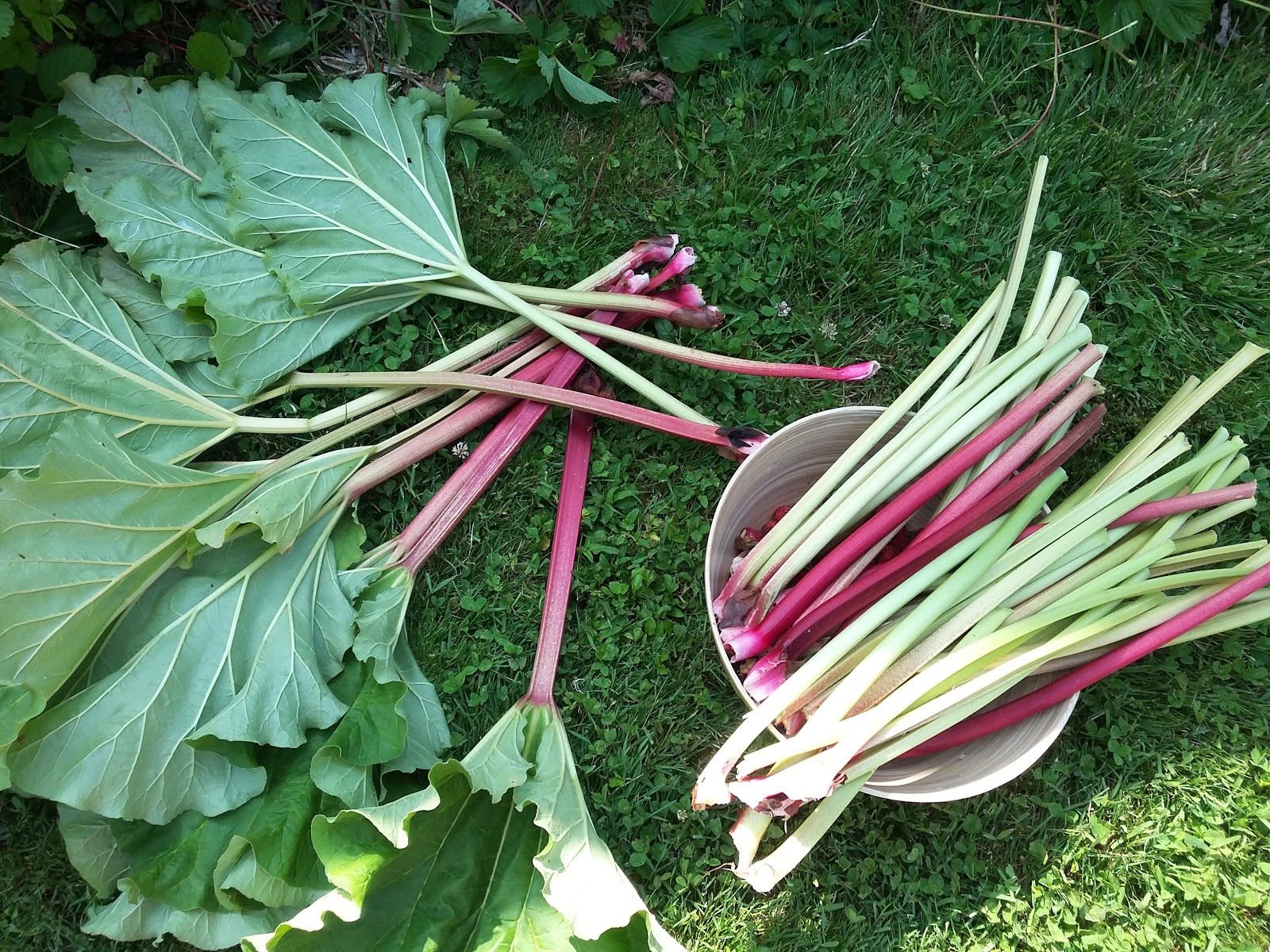The horizontal photograph captures a recently harvested strawberry rhubarb plant, with its stalks and leaves prominently displayed. On the left side of the image, a pile of uprooted rhubarb stalks lies scattered over a bed of grass and clover. The stalks range in color from pale green to a subtle pink, each ending in knobby, textured roots that curve where they were pulled from the soil. The leaves, characterized by their prominent veins, are mostly turned upside down, showcasing the intricate vein patterns.

Adjacent to the pile is a white bucket, partially filled with additional rhubarb stalks. Some of the stalks rest on the rim, while others are tucked inside, displaying a spectrum of hues from light green to dark pink. The bucket is viewed from above, allowing a clear look at its interior. Sunlight casts a gentle highlight on the lower right corner of the image, illuminating some of the stalks in the bucket and the bottom leaves in the pile, adding a touch of warmth to the scene.